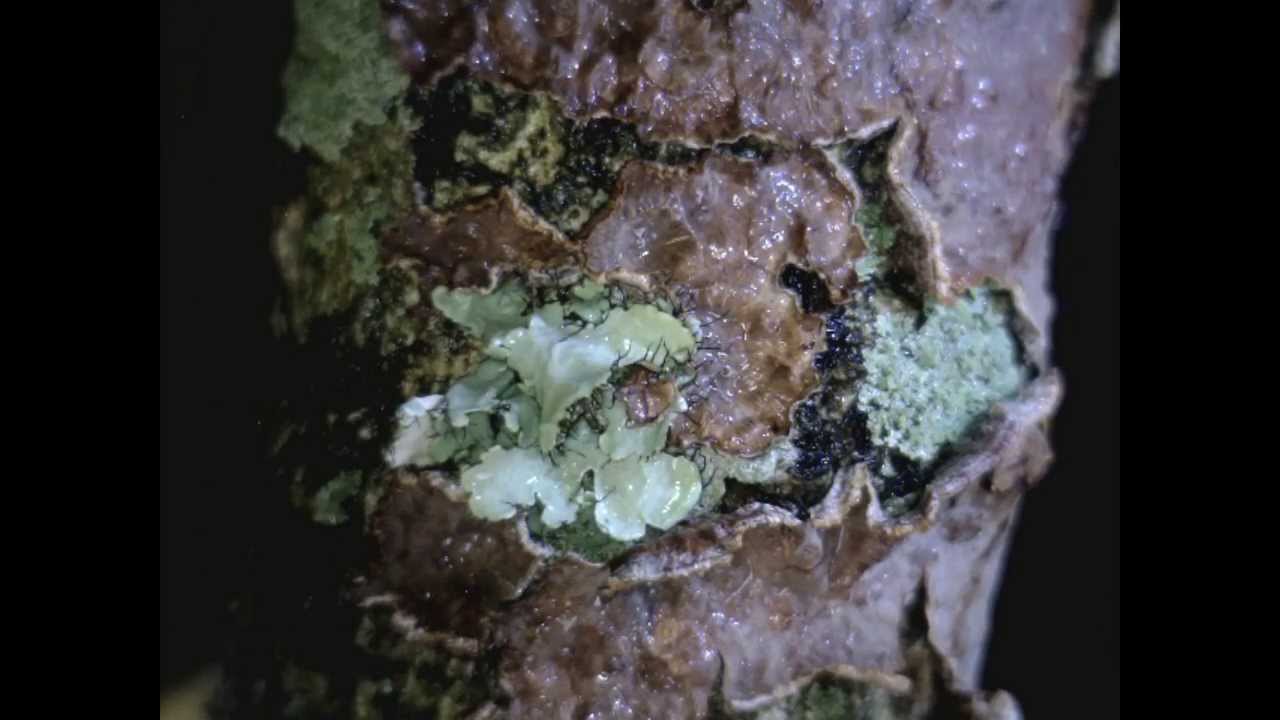This close-up photograph features an extremely grotesque and slimy-looking object likely of vegetal origin, possibly a mold-infested tree trunk. The background is pitch black, which accentuates the object’s unsettling appearance. The trunk, composed of brown, peeling bark, is covered in a clear, cloudy, and mucous-like substance that looks wet and repulsive. Green fungal growths resembling small leaves or mushrooms sprout from various points, particularly on the top right, top left, and center of the trunk. The green growths vary in size, with some minuscule and others larger, almost broccoli-like in appearance. Mixed within the bark's crevices are black seed-like elements, adding to the overall grotesque texture. Moist, silver-gray shiny flakes can be observed near the lower left center, interspersed among the brown, slimy masses that seem to peel off the trunk. The image's left and right borders are black, framing this detailed and disgusting close-up of nature's decay.